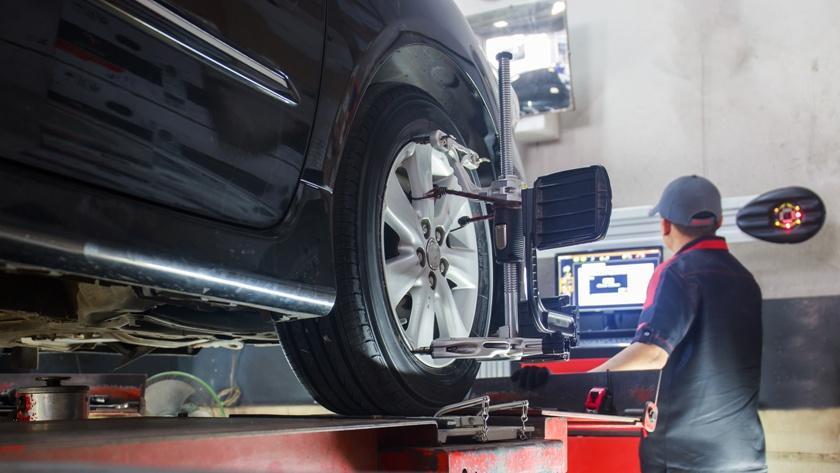In this detailed photograph taken inside an automotive shop, a dark-colored sedan, likely black, is elevated on a red lift so that its wheels are around eye height. Attached to the front wheel on the passenger side is a piece of equipment, possibly for diagnostics or testing. Standing in front of the car is a technician with his back to the camera. He is wearing a dark gray baseball cap, and a blue short-sleeved shirt with a red stripe along the collar, intently gazing at a computer screen, potentially monitoring the diagnostics. The facility appears clean and professional, characterized by concrete walls that have a slightly dingy appearance. The image captures a moment of focused work in what seems to be a well-equipped repair or testing shop.